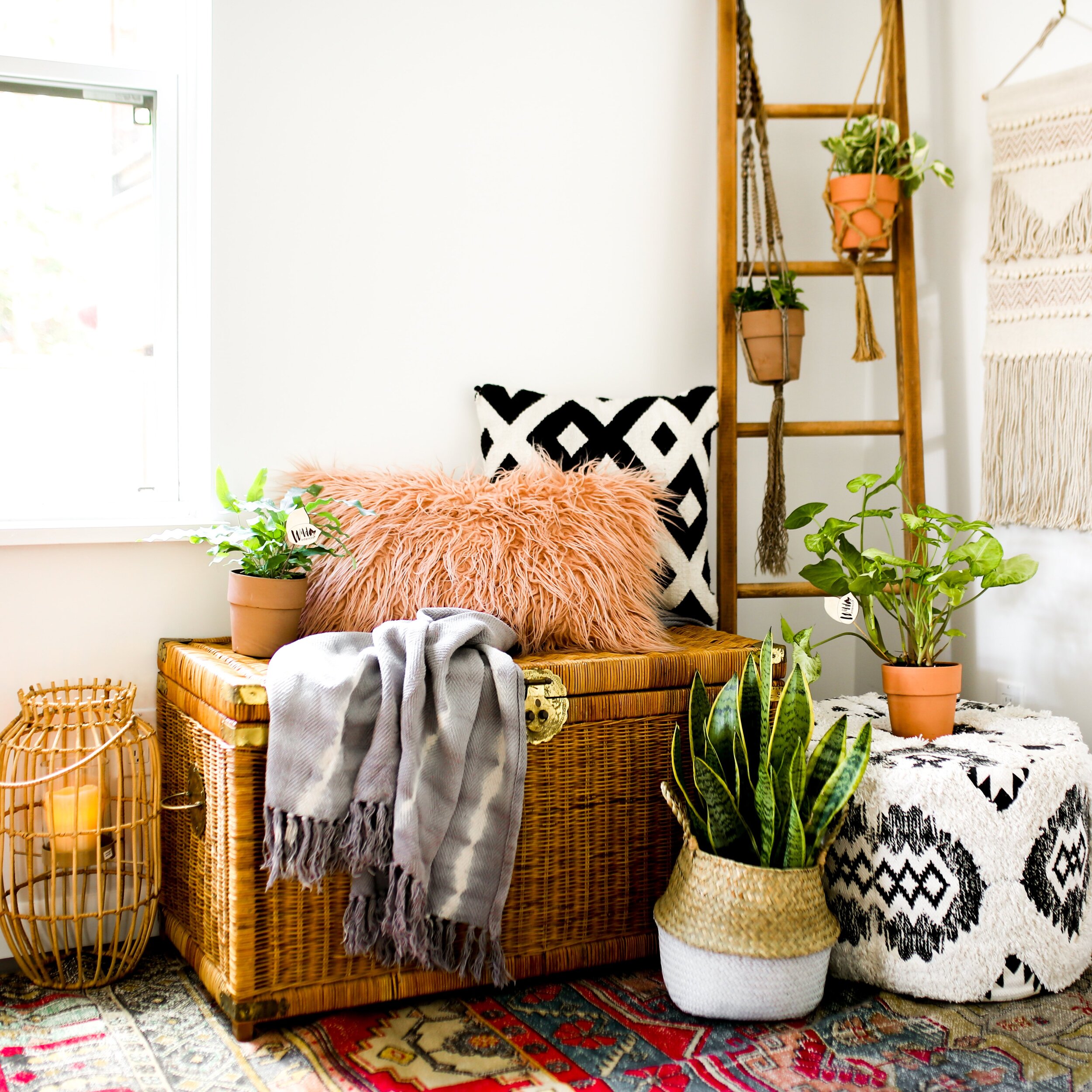This is a detailed close-up view of a cozy, boho-style corner in a room. In the backdrop, there's a plain white wall with a window on the left that has no coverings, allowing bright white light to illuminate the space. Central to the scene is a large wooden ladder-style plant stand with two hanging terracotta planters suspended by ropes, each containing a different type of green plant. Below the ladder stands a small black-and-white patterned ottoman topped with another terracotta planter.

Adjacent to the ladder is a woven wicker chest featuring a vintage gold hinge. Draped over the chest is a gray blanket, and leaning against the back is a pair of plush pillows: a fluffy pinkish-orange one and a black-and-white geometric one. On the left corner of the chest sits yet another terracotta planter. 

To the left of the chest, directly beneath the window, there is a tall, round wicker candle holder with a metal hanger, complementing the rustic nature of the room. In front of the chest, there's a white and wicker plant basket with wicker handles containing a vibrant snake plant.

The floor is adorned with colorful oriental rugs in shades of red and gold, adding to the warm, inviting atmosphere. Overall, the scene is meticulously staged to reflect a bohemian aesthetic with vintage elements, enriched by an array of green plants and textured decor pieces.